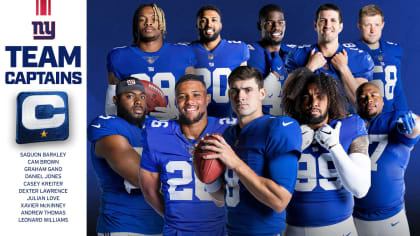This promotional photograph features ten football players from the New York Giants NFL team, organized into two rows with the bottom row positioned foremost. The players are clad in blue jerseys with white lettering. Among them, there are seven black men and three white men. In the middle of the front row, a player is holding a football, posed as if ready to throw. Flanking him are two larger black players. Some of the players have their arms crossed, one is pointing at the camera, and two are gripping the neck of their jerseys from the front.

On the left-hand side of the image, the New York Giants logo, an "NY," is prominently displayed above the text "Team Captains," which features a blue logo with a "C" and a star. The names listed below the logo include Saquon Barkley, Cam Brown, Graham Gano, Daniel Jones, Casey Kreider, Dexter Lawrence, Julian Love, Xavier McKinney, Andrew Thomas, and Leonard Williams.